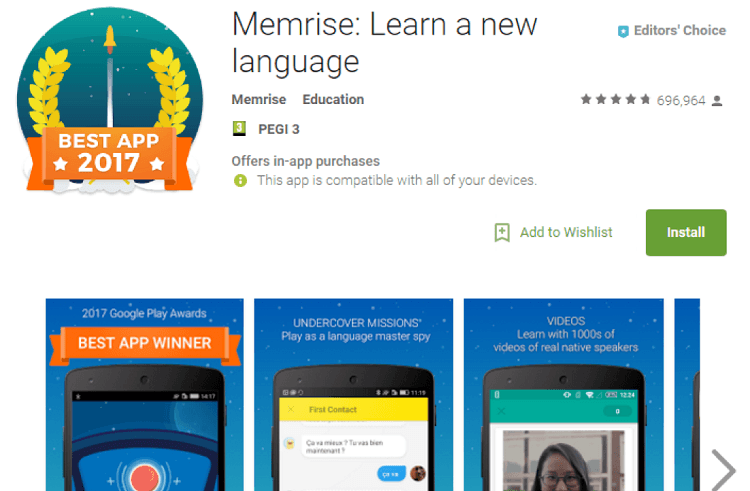Screenshot of a webpage displaying an award-winning app. The top-left corner showcases the "Best App of 2017" award, depicted as a snow globe with a night sky filled with stars and a little rocket ascending to the top. To the right of this award image, the text reads "Memorize New: Learn a New Language," with an "Editor's Choice" badge featured in the upper right corner. Below this, the app is categorized under "Memorize Education" and indicates it offers in-app purchases and is compatible with all devices. A significant number of reviews are noted, with 696,964 people having given feedback. Buttons for "Add to Wishlist" and "Install" are also visible. Below these details, there are three preview images, each in blue boxes. The first image states "2017 Google Play Awards Best App Winner"; the second promotes "Undiscover: Undercover Musicians Play as a Language Master Spy"; and the third highlights "Videos: Learn with Thousands of Videos of Real Native Speakers." An arrow on the right indicates the option to scroll through more images.